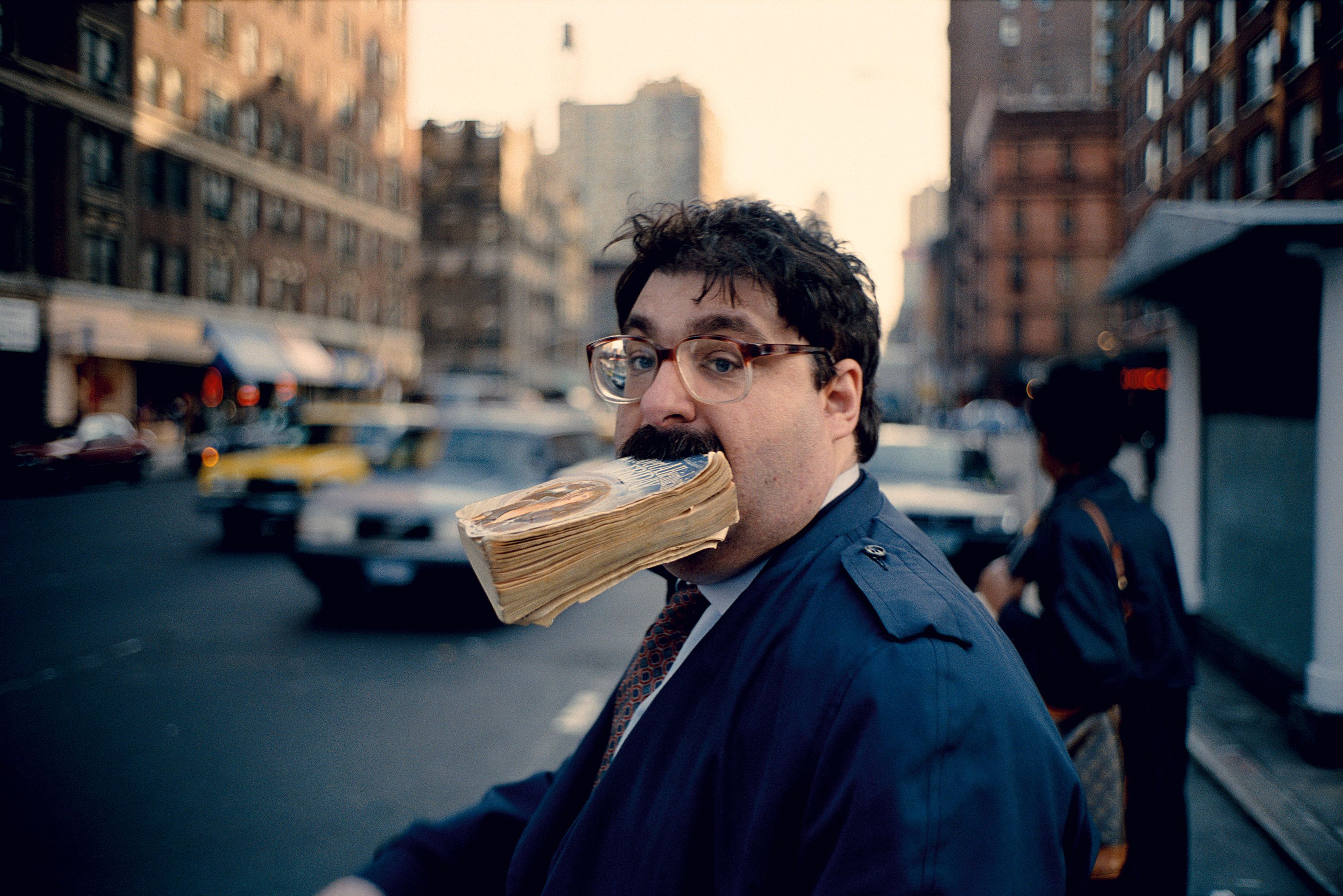In this urban street scene, a man with disheveled, dark hair stands at the forefront, gazing directly into the camera. He sports a very thick mustache and thick-framed glasses. A dark blue jacket with a distinct button flap on the shoulder covers his white collared shirt and black-accented tie. Unconventionally, he holds a book in his mouth, which appears to be an older novel, perhaps even a romance. The bustling city backdrop reveals a line of cars, including a distinctly identifiable taxi cab, indicative of a location like New York. Behind him, another person can be seen wearing a hat and a shoulder bag, also dressed in a dark jacket, adding to the layered, dynamic street composition.